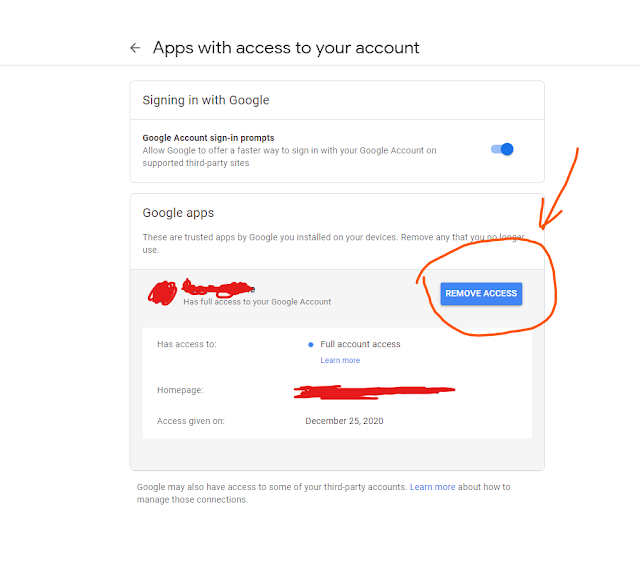The image depicts a sign-in page formatted for a mobile or tablet device, aimed at managing third-party app access to a Google account. At the top-left corner, there is a back arrow icon, providing easy navigation. The page's header is prominently displayed with the text "Apps with access to your account" in black against a white background.

The primary section of the page features a rectangular box where users can manage their account settings. At the top of this box, bold text reads "Sign in with Google," followed by a message explaining that "Google's account sign-in prompts are turned on. Allow Google to offer a faster way to sign in with your Google account on supported third-party sites."

Further down, the section is titled "Google Apps," indicating the specific focus on trusted applications by Google installed on the user's devices. The text advises users to "remove any that you no longer use."

Within this section, there is another rectangle bordered in gray, which contains a blue "Remove Access" button. This button is highlighted with a red circle and an arrow pointing to it for emphasis. Notably, the name of the app and its home page within this box have been scribbled out in red, presumably to protect privacy.

Overall, the image is a detailed representation of managing app access on a Google account through a user-friendly interface designed for mobile or tablet use.